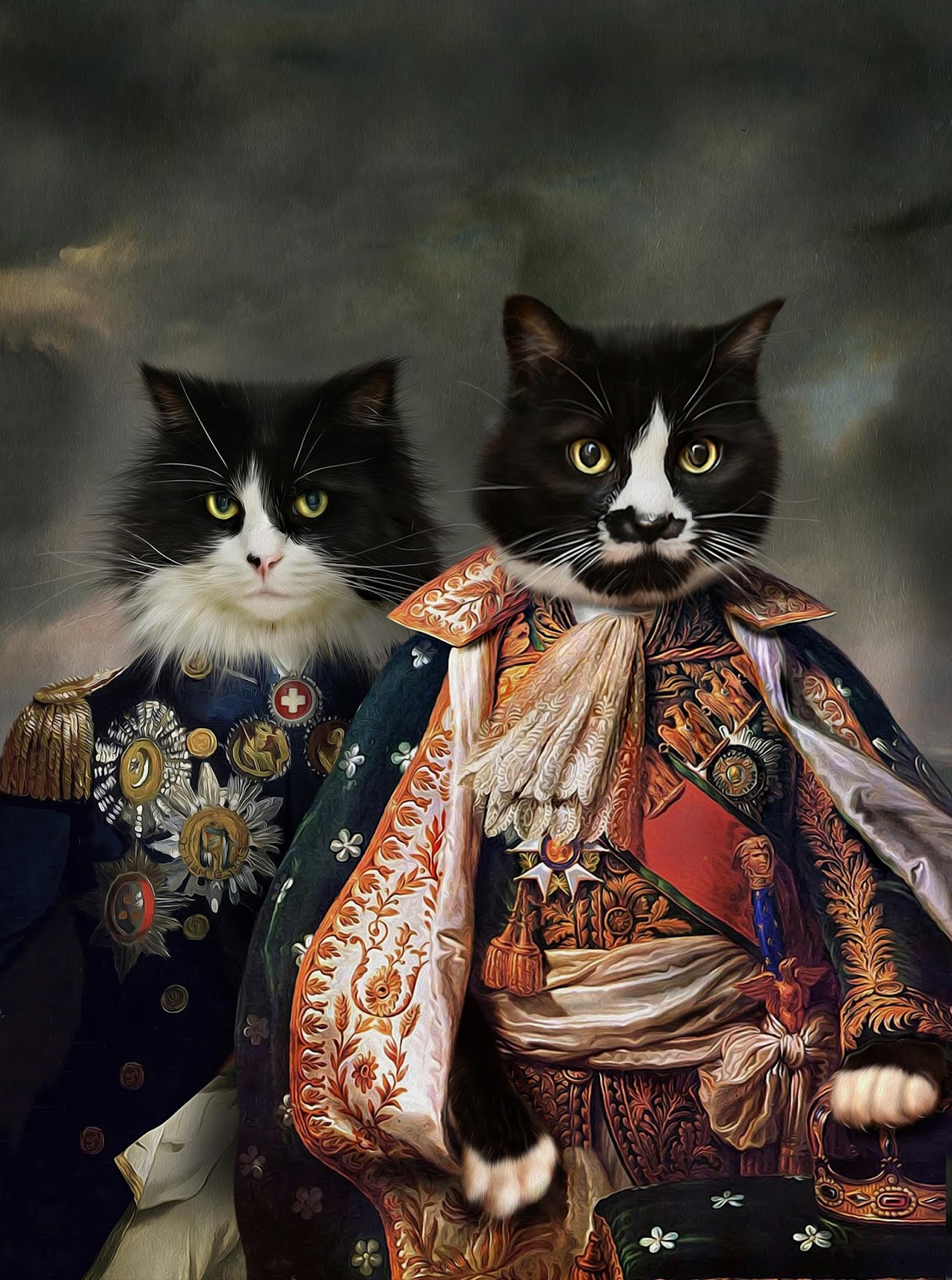In this vertically oriented, rectangular close-up portrait photograph, we see an adorably whimsical scene featuring two tuxedo cats, both adorned in regal, king-and-queen-style attire. These cats, characterized by their distinctive black and white "tuxedo" markings, are posing side by side, creating a captivating and endearing image.

The tuxedo cat on the right is dressed in an opulent costume, composed of rich gold and black fabrics, adorned with intricate embellishments including metals, feathers, and stars. The array of details creates a lavish and authoritative presence, further emphasized by the cat's posture as it elegantly holds its front paw over a golden crown, symbolizing its royal status.

To the left, the second tuxedo cat mirrors the grandeur of its companion, wearing an equally elaborate outfit. This costume similarly features metallic adornments and a luxurious gold embellishment on its left shoulder. Both cats share strikingly beautiful yellow eyes, their large black pupils adding a touch of mystique to their royal personas.

The photograph captures an amusing and charming tableau, blending the whimsical nature of feline grace with the majestic grandeur of royal attire, making it a delightful and detailed portrayal of these tuxedo cats in their regal best.